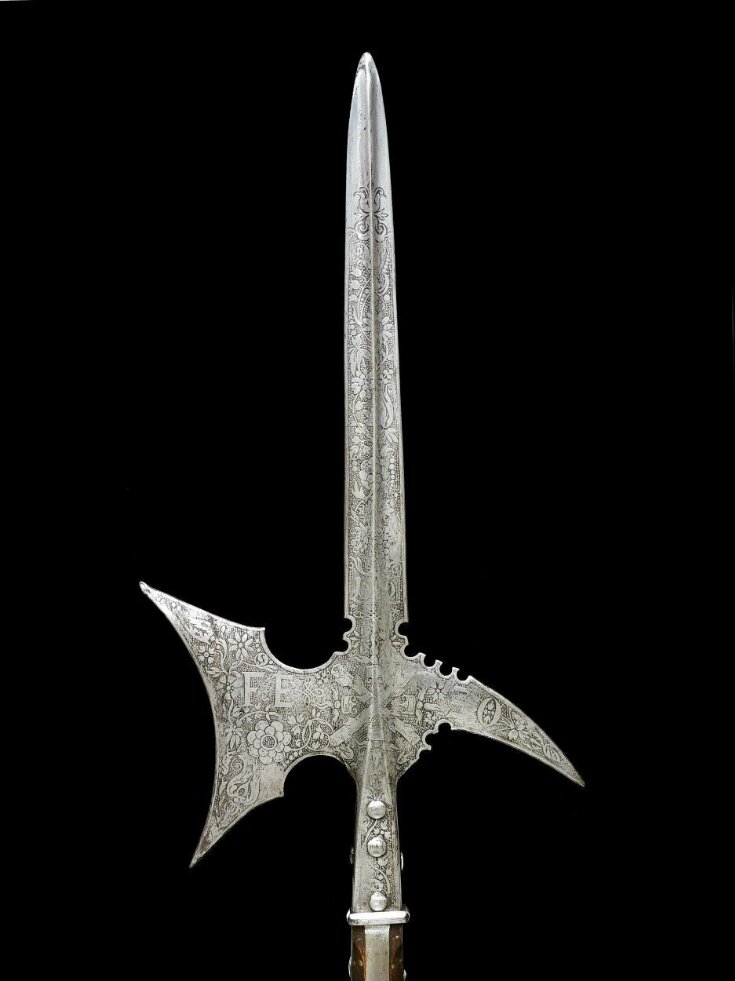The image presents a medieval-era weapon prominently displayed against a solid black background. The object is a finely crafted sword, featuring a silver blade with intricate engravings spanning approximately three-quarters of its length, adorned with floral patterns and vines, though the tip remains unadorned. The sword also exhibits a distinctive fin just before the handle, which is itself an elegant combination of wood and silver. Etched onto the weapon near the hilt are the letters "F" and "E," potentially signifying a maker's mark or an identifying emblem. The scene is illuminated with natural lighting, revealing every detail of the well-preserved weapon, suggesting its status as a prized museum artifact. The clarity and brightness of the image highlight the sharpness and potential lethality of the blade, underscoring its historical significance and formidable design.